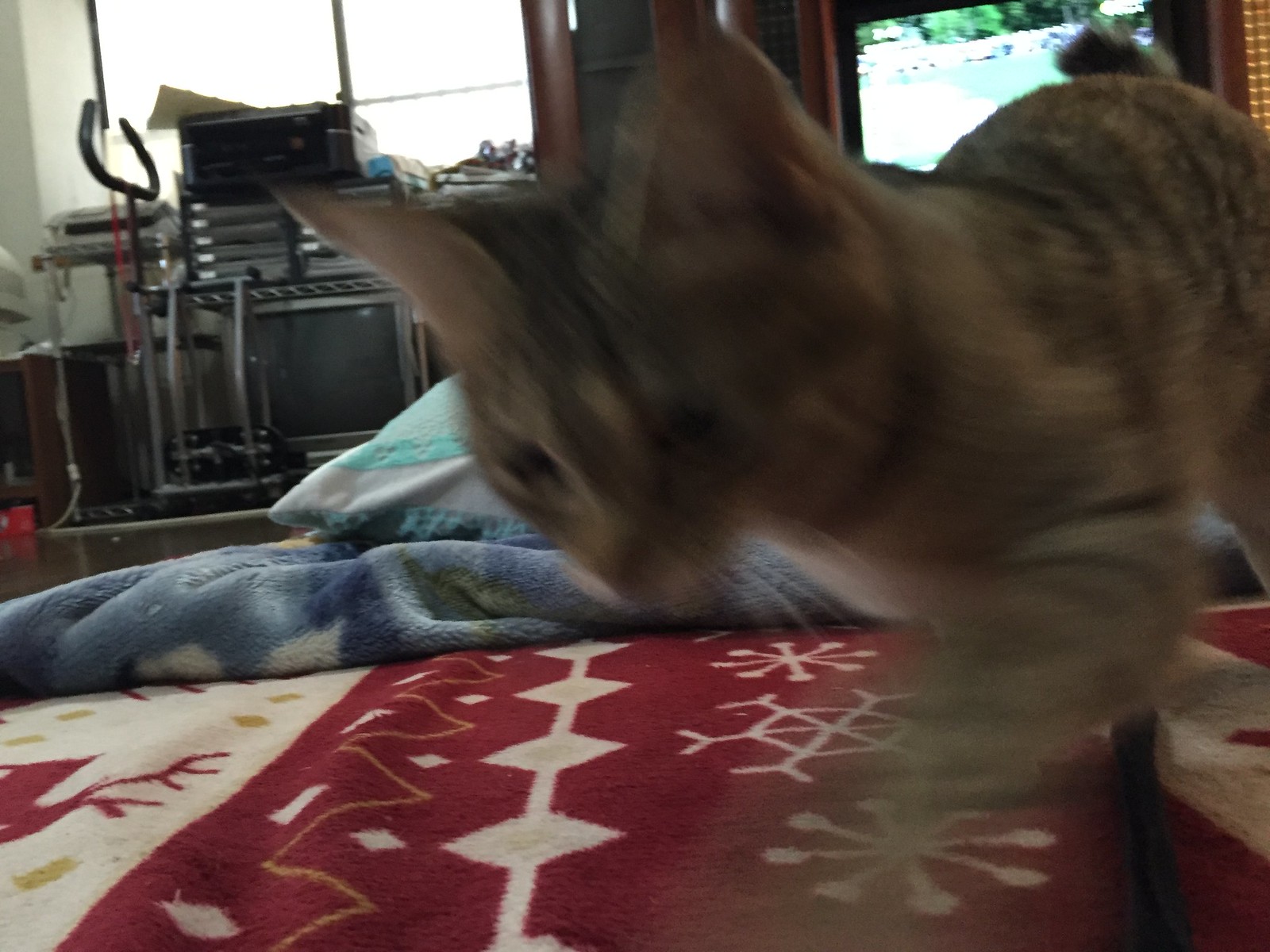In the foreground of the image, a medium to small-sized cat occupies the central focus, albeit slightly out of focus. The feline features a coat with a rich tapestry of brown fur adorned with distinctive black or darker-colored stripes, interspersed with patches of lighter hues. The cat's eyes appear dark, partially obscured by poor lighting, which casts shadows over its face. The ears are prominent and pointy.

The cat sits upon a festive Christmas-patterned carpet displaying an intricate design of red reindeer and white snowflakes set against a red background. The carpet also features a white-lined band decorated with white diamonds, accompanied by a yellow line encircled by smaller white diamonds.

In the background, a television screen emits a faint glow, indicating it is turned on. There is also a window through which daylight filters, suggesting an overcast or gray day. Additional elements in the room include another television that is turned off and various unidentified objects cluttering the corner, adding to the scene's domestic ambiance.